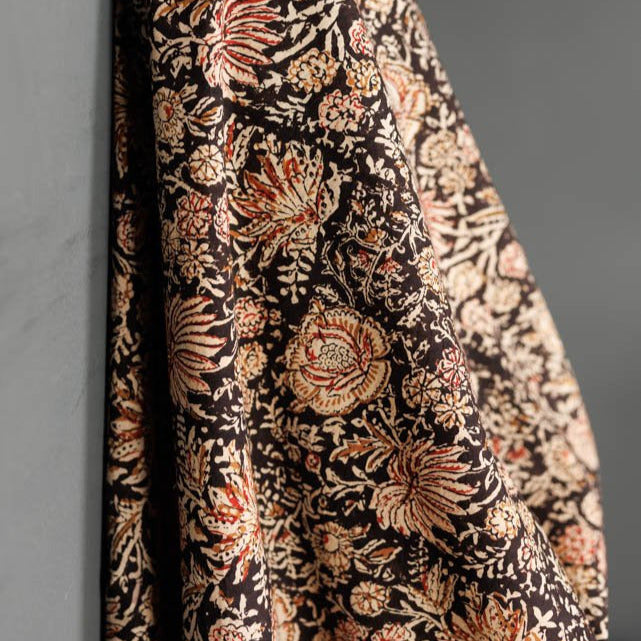This detailed close-up image showcases a piece of fabric laid flat against a gray background, viewed vertically. The fabric features a predominantly black backdrop adorned with intricate floral patterns. Cream-colored flowers with tips tinged in red and orange dot the landscape, sharing space with a singular round beige flower, meticulously outlined in brown and detailed with brown lines along its edges. A vibrant red center adds a pop of color to this standout bloom. Interspersed among the flowers are delicate white leaves, adding to the intricate design. On the left side, the fabric is folded and sewn over to create a visible edge, hinting at the construction of a possible skull cap. This edge reveals two layers of black material within, offering a peek at the complex craftsmanship behind the fabric’s creation.